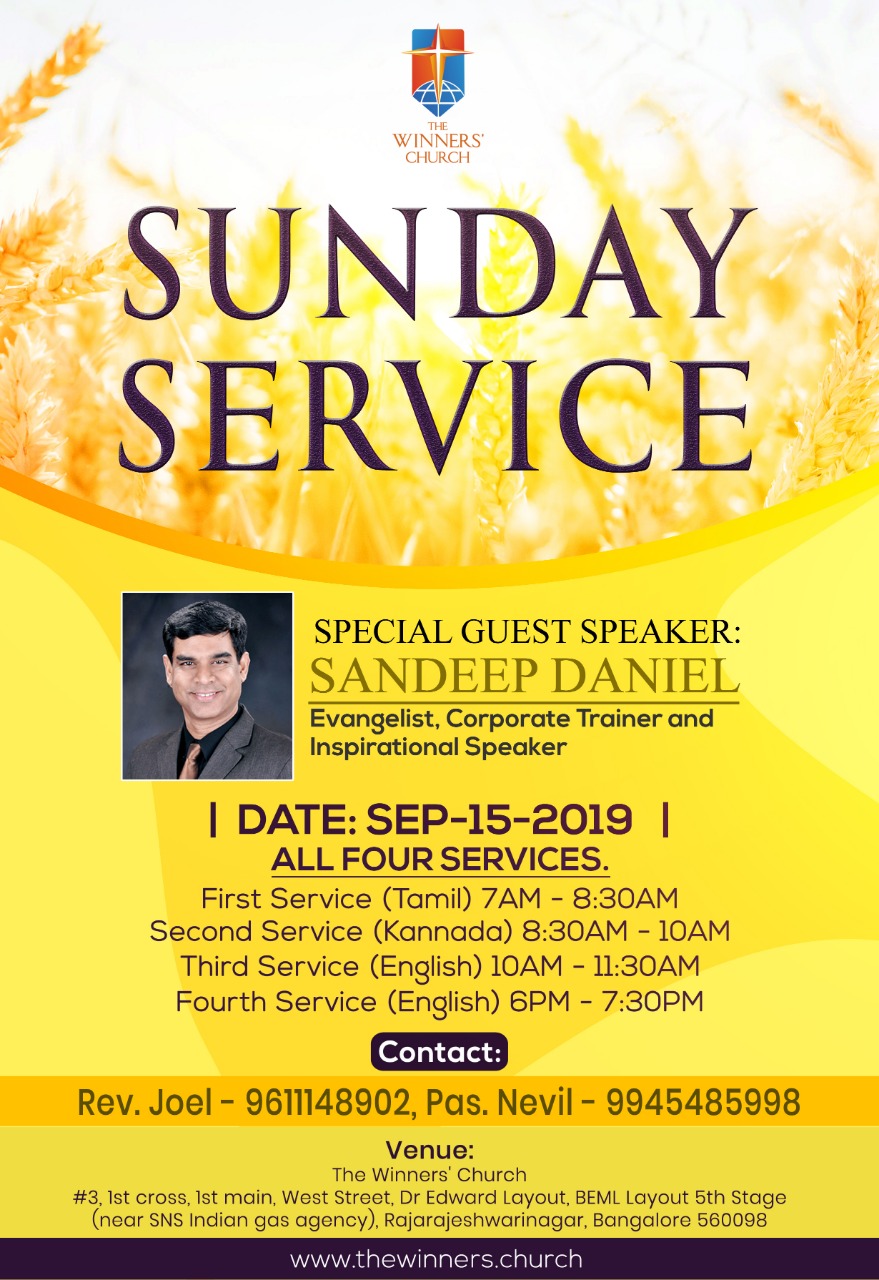An advertisement poster for an event at The Winner's Church, prominently featuring a dynamic design with a mainly yellow background. At the very top, there is a distinctive logo in red and orange adorned with a gold cross, followed by "The Winner's Church" in elegant gold letters against a subtly textured, grainy white backdrop. Beneath this, bold black text announces "Sunday Service" with an orange line fading into yellow below it, further enhancing the visual appeal. The lower section transitions to different shades of yellow and prominently showcases a headshot of the special guest speaker, Sandeep Daniel. He has dark black hair, is smiling with his teeth just visible, and is clad in a gray suit, black shirt, and an orange or gold tie. Adjacent to his image, the text states: "Special Guest Speaker Sandeep Daniel, Evangelist, Corporate Trainer, and Inspirational Speaker." Below this, details of the event are meticulously listed, highlighting the date as September 15, 2019, and outlining all four service timings: First Service in Tamil, 7:00 AM to 8:30 AM; Second Service in Kannada, 8:30 AM to 10:00 AM; Third Service in English, 10:00 AM to 11:30 AM; and Fourth Service in English, 6:00 PM to 7:30 PM. The contact section features details for Reverend Joel at 9611148902 and Pastor Neville at 9945485998. Venue information specifies The Winner's Church, situated at Number 3, First Cross, First Main West Street, Dr. Edward Layout, BEML Layout Fifth Stage, near S&S Indian Gas Agency, Bangalore 560098. Concluding the poster is a black bar at the bottom displaying "www.thewinterschurch" in white text.